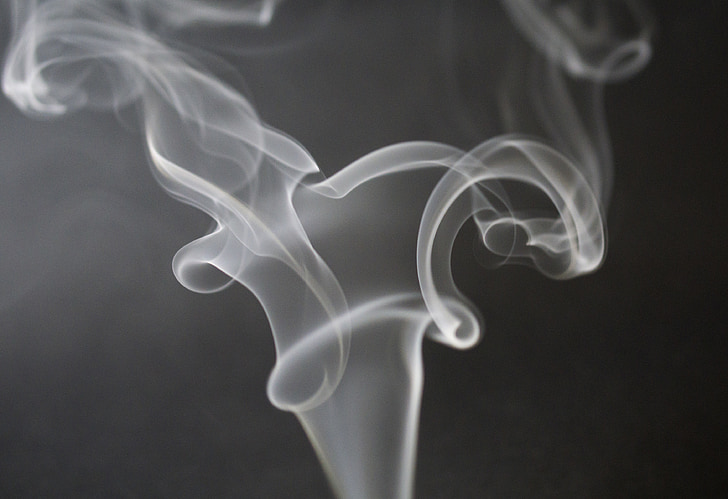This close-up, artistic black-and-white photograph captures the elegant and delicate movement of thin, wispy smoke rising from a narrow point at the bottom center of the image. The smoke, which appears white and various shades of gray, spirals and swirls as it ascends, filling almost the entire width of the horizontally-oriented rectangle at the top. The background shifts from dark gray, almost black on the right, to a slightly lighter gray on the left, creating a striking contrast that emphasizes the subtlety of the smoke's intricate curls and layers. These smoke plumes, which evoke the remnants of a puff of cigarette or similar light smoke source, form a broad, undulating U shape with multiple waves and swooping motions, conveying a sense of grace and fluidity. The photograph is devoid of any other elements, highlighting its minimalist and artistic nature.